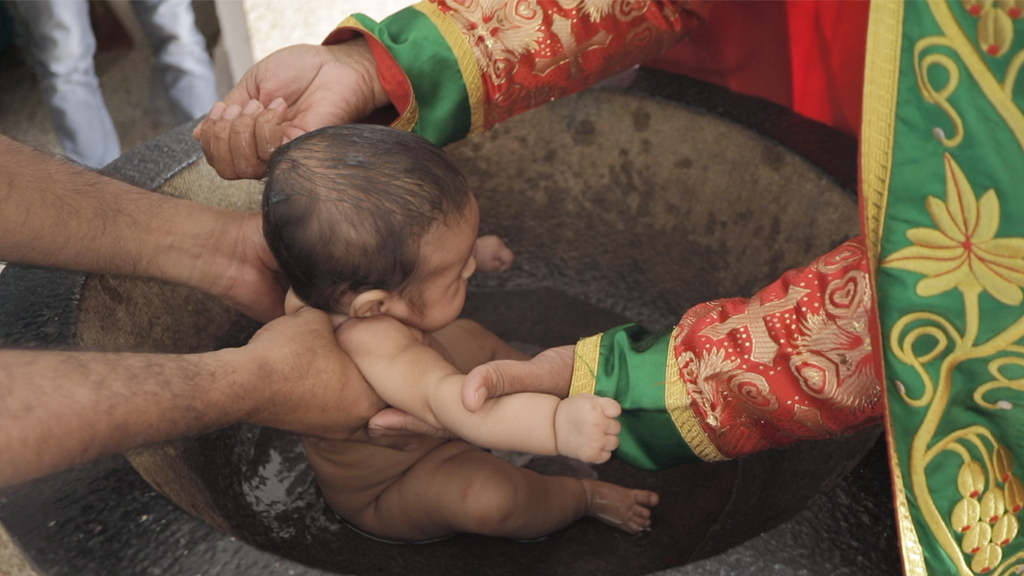In this image, a newborn baby with dark black hair is being baptized. The infant, naked and facing towards the right, is being supported by two pairs of hands. The hands on the left are hairy and belong to a man, while the arms coming from the right, likely those of a priest, are adorned in an elaborate robe featuring green, red, and gold patterns with leaf motifs and gold embroidery. The individual in the robe appears to be performing the baptism as they cupped water, ready to pour it over the baby. The baby is being held over a large, round, stone container filled with brown, murky water, indicating the event is taking place during the day, possibly near an open doorway. Both individuals holding the baby are men, although their faces are not visible in the picture. The setting and attire emphasize the ceremonial and religious significance of the moment.